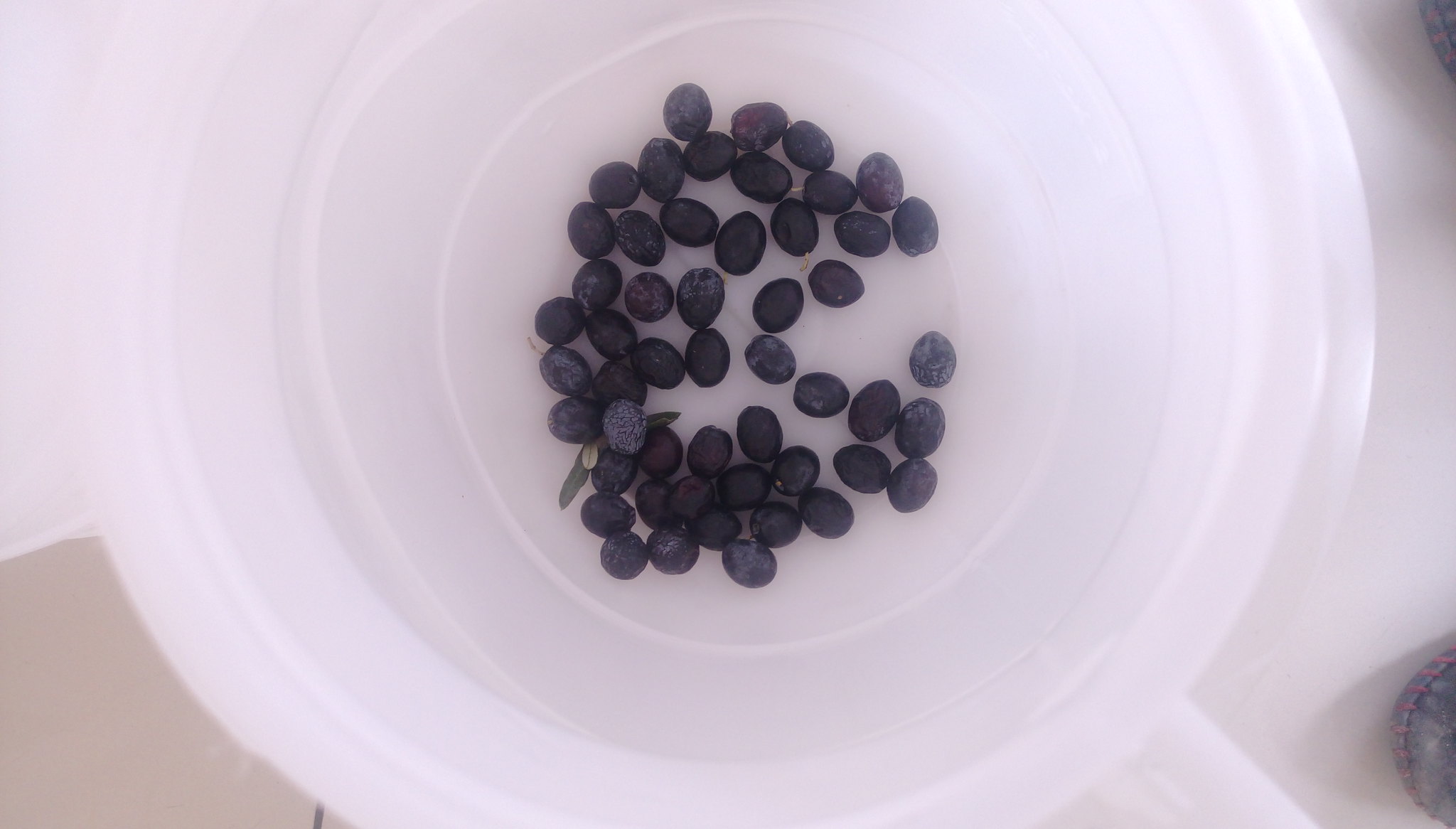This is a detailed photograph looking directly down into a white plastic bowl with a slightly translucent surface, allowing some light to pass through. The bowl contains approximately 20 to 30 small, dark blue to almost black, oblong-shaped berries, resembling either small grapes or an unidentified type of fruit. Some of these berries display a light, powdery speckling, similar to the natural bloom found on fresh grapes. Mixed among the berries, in the bottom left corner, is a small green twig, suggesting the fruit is unwashed and freshly picked. The background of the image consists of a white surface, possibly a countertop, and additional indistinct white objects, which could be a wall, tile, or perhaps an appliance. The scene gives an impression of simplicity and natural freshness.